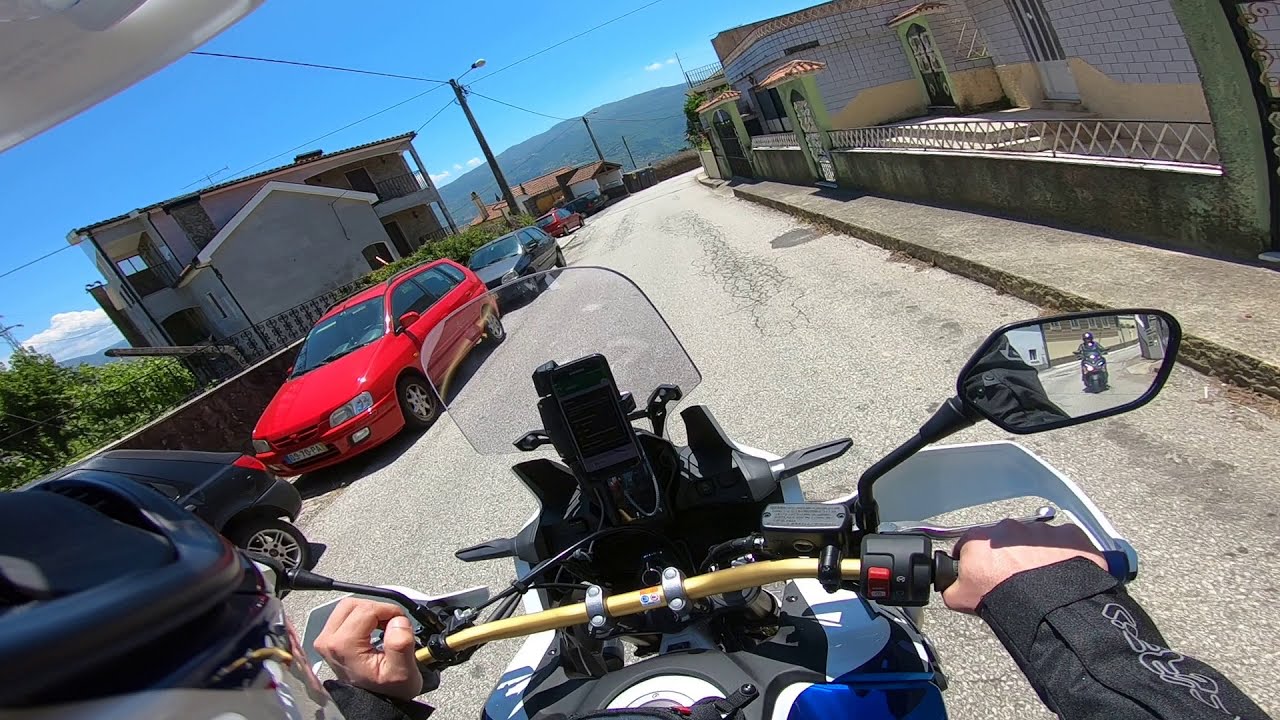This image captures a first-person perspective of a man riding a motorcycle down a narrow, private road, seemingly in a European setting. The man is wearing a black motorcycle jacket, visible on his arms as he grips the handlebars, with the right hand clutching the throttle. The motorcycle's dashboard and controls, including the clutch and center console with a small plastic visor, are clearly visible. The rear-view mirror on the right side of the bike reveals another motorcyclist trailing behind him.

To the left of the road, a small stone wall and several parked cars can be seen, including a red car and multiple black cars. On the right side, there are houses, one notably made of white bricks. The clean, blue sky above is dotted with puffy white clouds, while a hill or mountaintop range provides a scenic backdrop. The road itself, though somewhat well-maintained, shows a few cracks, adding to the sense of a quiet, rustic environment.